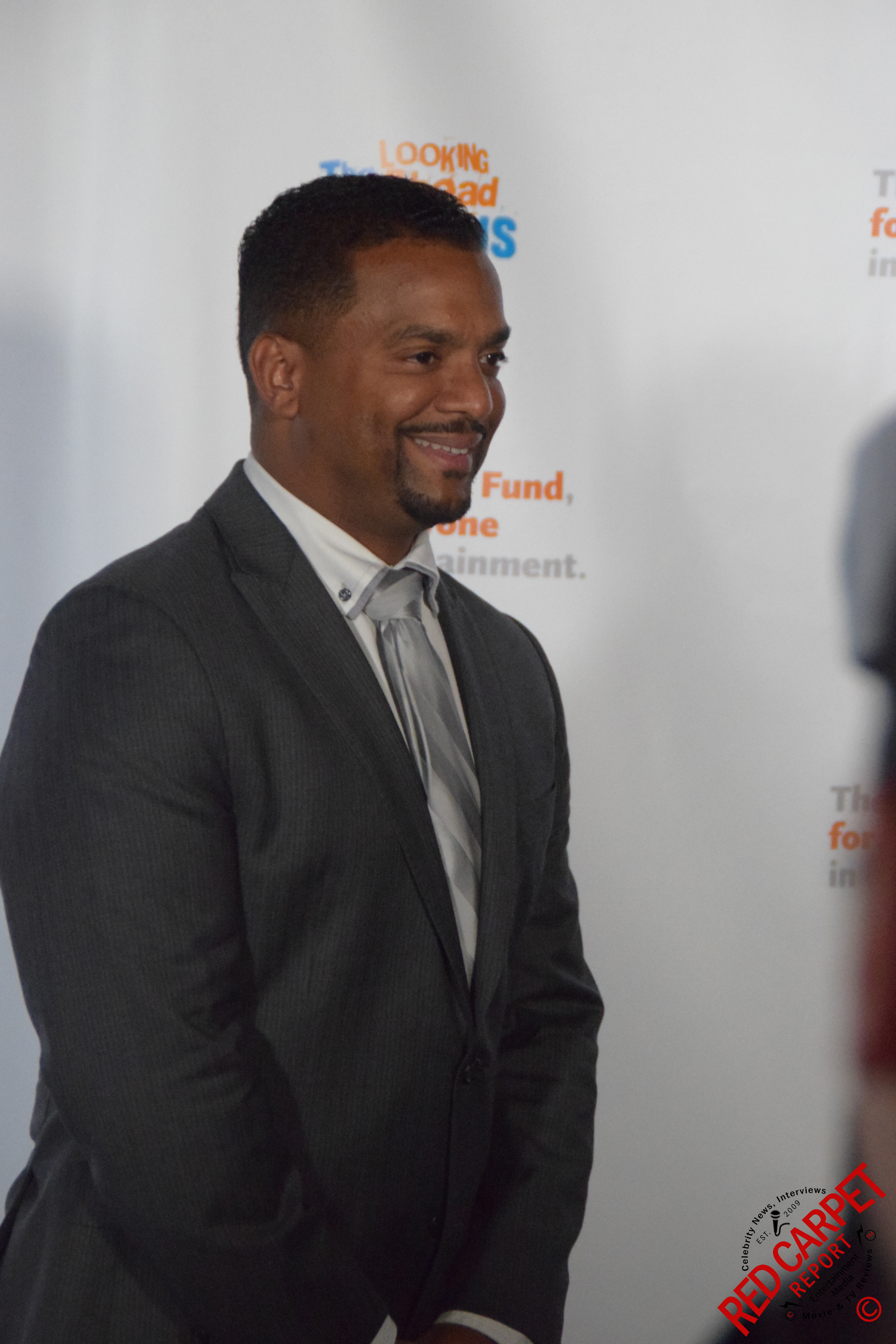The image showcases a smiling African-American man, identified as Alfonso Ribeiro—known from "The Fresh Prince of Bel-Air" and as the host of "America’s Funniest Home Videos." He is dressed in a dark gray suit, a white button-down shirt with dark buttons, and a silvery striped tie. His mustache and goatee complement his cheerful expression as he looks towards the left. The backdrop features partially obscured orange and blue lettering, seemingly hinting at an event's name, with “Looking Fund 1” partially visible. In the bottom right corner, a logo and the text “Red Carpet Report, Celebrity News Interviews” are seen, suggesting a formal event atmosphere. Shadows from the event's lighting cast subtly on the backdrop, enhancing the professional setting.